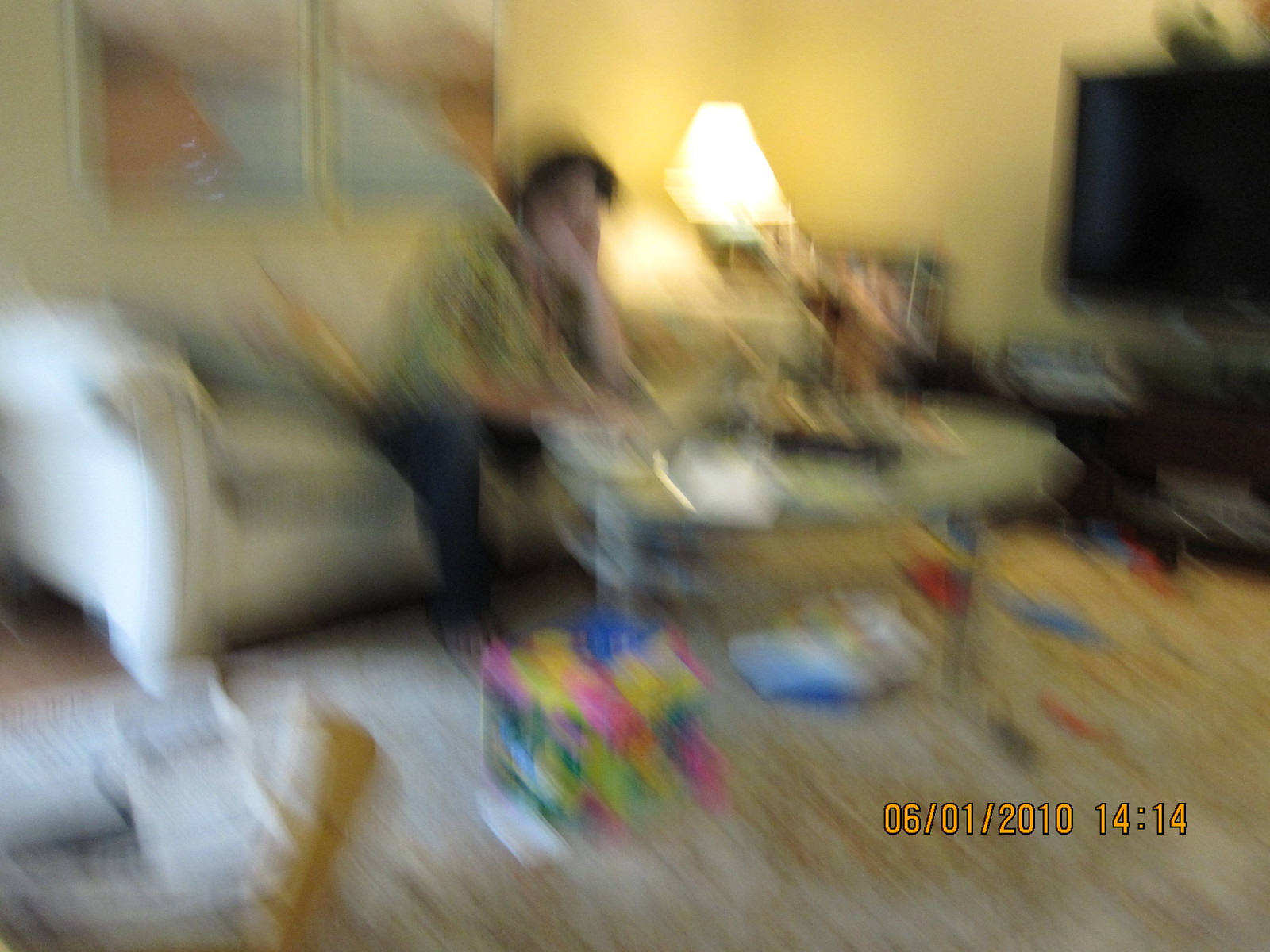In this exceptionally blurry photograph, dated June 1, 2010, at 14:14, a man is seated in his living room. The individual, who appears to have a larger frame and is of Caucasian descent, is positioned centrally on a cream-colored sofa. He is dressed in jeans and a short-sleeved, printed shirt with green and possibly brown patterns. He rests his left elbow on his left thigh, with his chin nestled in his hands. The man, sporting brown hair and glasses, gazes towards an undefined direction. 

Directly in front of him stands an oval-shaped glass coffee table set on a metal frame, cluttered with indiscernible items. To his left, there is a flat-screen TV, turned off, perched atop a dark wooden console. Behind him, a lit lamp is stationed on a side table, casting a gentle glow in the corner of the room. The floor is scattered with what seems to be children's toys, strewn across a cream-colored carpet.